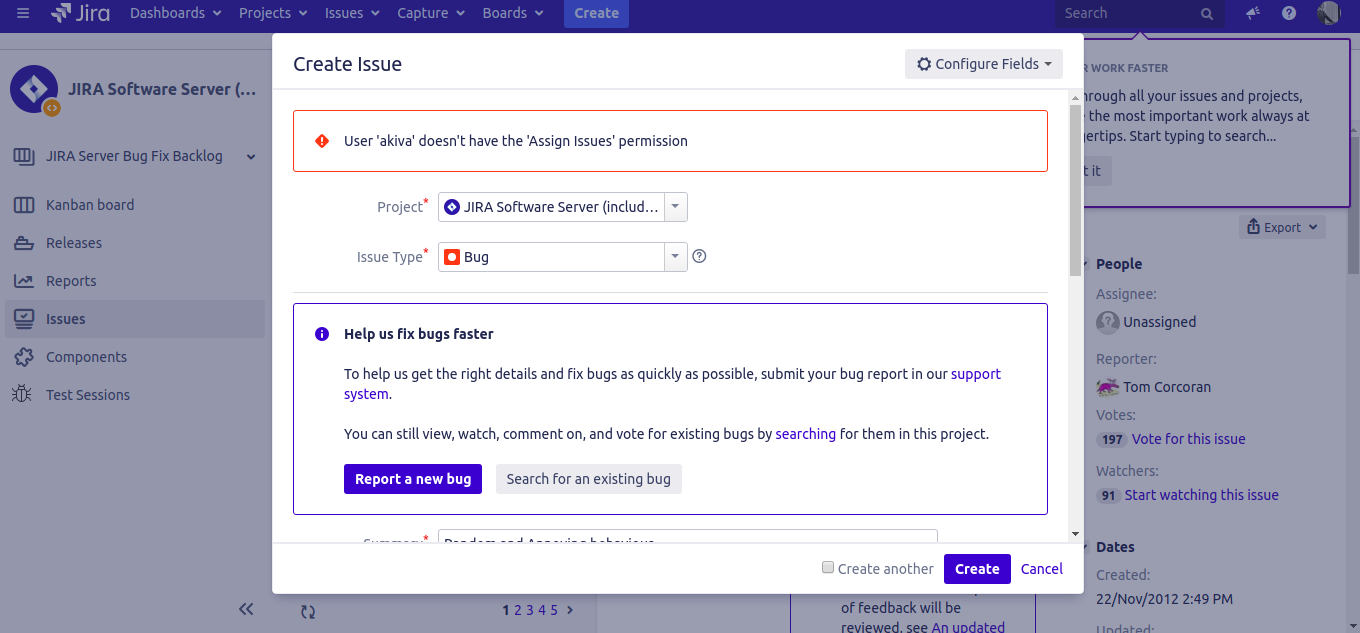In this screenshot, we see a prominent white rectangular box at the top of a partially grayed-out screen. In the upper left corner of the white box, there is black text that reads "Create Issue." To the right, there is a light gray box labeled "Configure Fields." Below that, there's a red-outlined box containing a message: "User Akiva doesn't have the permission to assign issues."

Further down, there is a dropdown menu labeled "Project" with "JIRA Software Server" selected. Directly underneath, there’s another dropdown menu titled "Issue Type," with "Bug" selected. Below this section is a blue-outlined rectangle featuring black text: "Help us fix bugs faster. To help us get the right details and fix bugs as quickly as possible, submit your bug report in our support system. You can still view, watch, comment on, and vote for existing bugs by searching for them in this project."

At the bottom of the screen, there are two buttons: a blue box labeled "Report a New Bug" and a white box labeled "Search for an Existing Bug." The interface aims to guide users on how to report and manage bug issues efficiently.